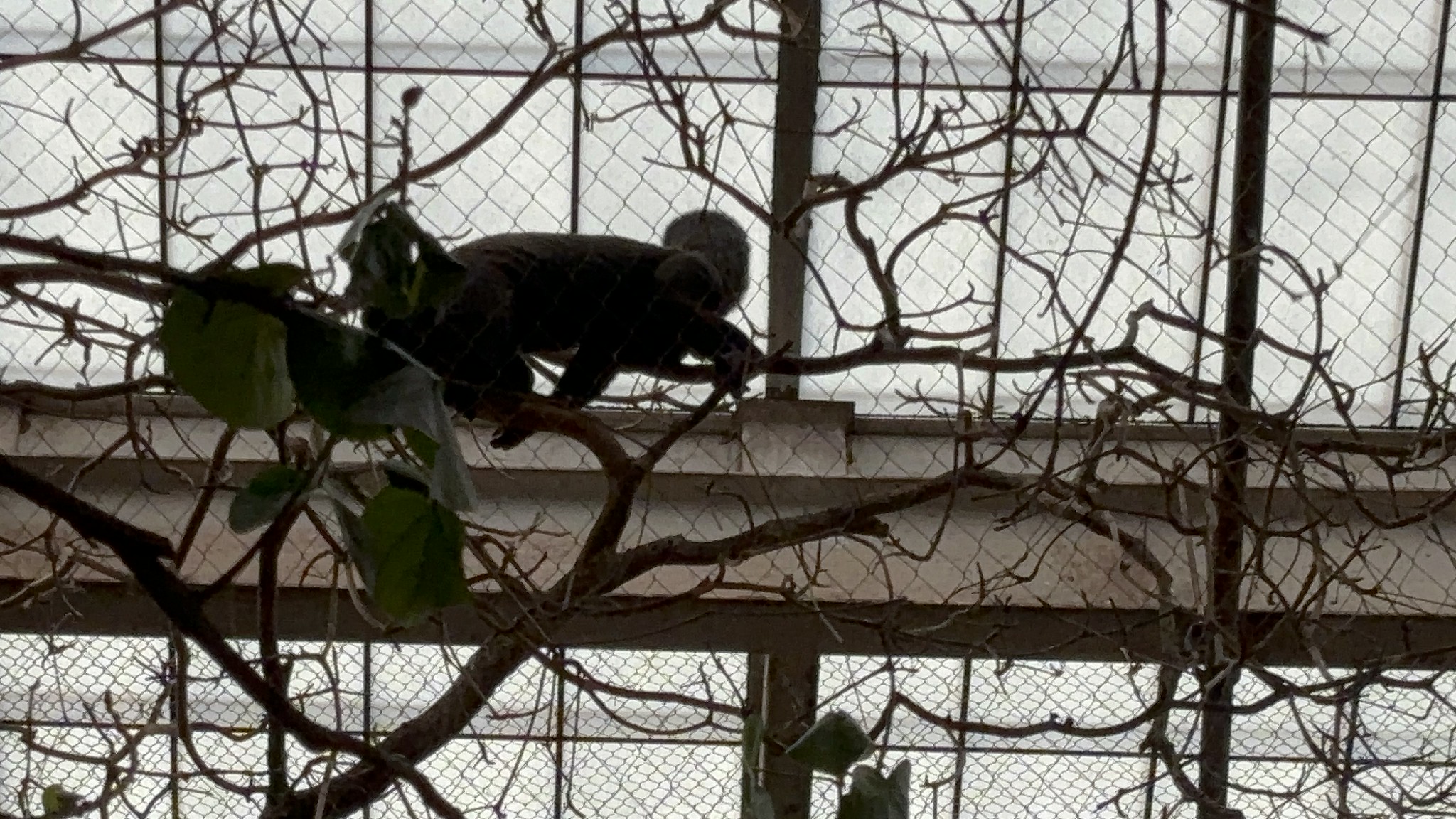In the indoor image, a small, dark black monkey is perched on top of a white metal rafter, its head raised close to a chain link fence that covers the frosted skylight above. The fence has a white cover allowing light to pass through, casting nuanced shadows around the scene. Metal bars of a darker color run across the rafter, partially enveloped in shadows. The majority of the rafter is obstructed by bare, green branches with very few leaves, some of which droop from the left side and a couple of leaves emerge centrally at the bottom. The background features smaller-holed chickenware fencing towards the bottom, and the overall color palette includes white, black, brown, green, and tan hues. The scene suggests the setting is within a zoo, emphasizing a contrast between the dimly lit interior and the illuminated cover above. The image captures the intricate interplay of light and shadow, giving it a slightly darker tone, thereby making finer details more elusive.